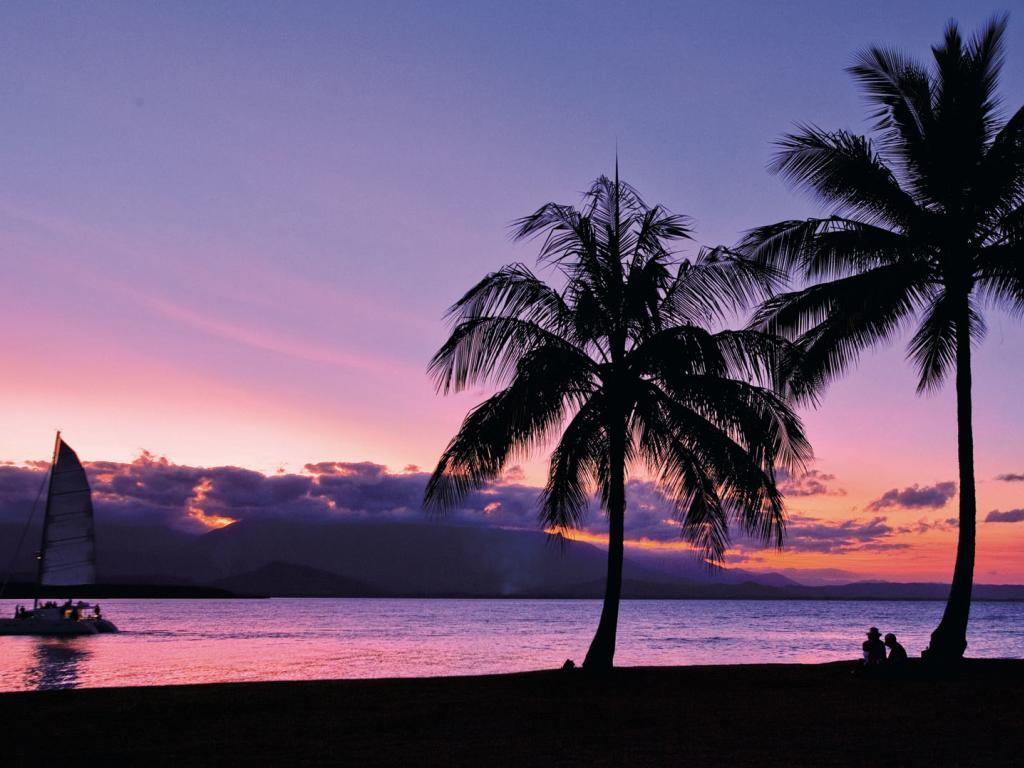In this awe-inspiring, tropical beach scene at dusk, the sun has just set, painting the sky in a mesmerizing blend of purple, orange, pink, and blue hues. The tranquil waters reflect these brilliant colors, creating a glassy, serene surface. In the foreground, two majestic palm trees stand tall, their silhouetted forms striking against the vibrant sky. Nestled near one of the palm trees are the shadows of two people, sitting and absorbing the peaceful, breathtaking view. A sailboat, also in shadow, glides silently along the water, adding to the sense of calm. Faint clouds linger on the horizon, above dark hills in the distance. The entire beach appears cloaked in darkness, with the sand hidden in the twilight, contributing to the scene's enchanting, almost mystical atmosphere, reminiscent of a Hawaiian paradise.